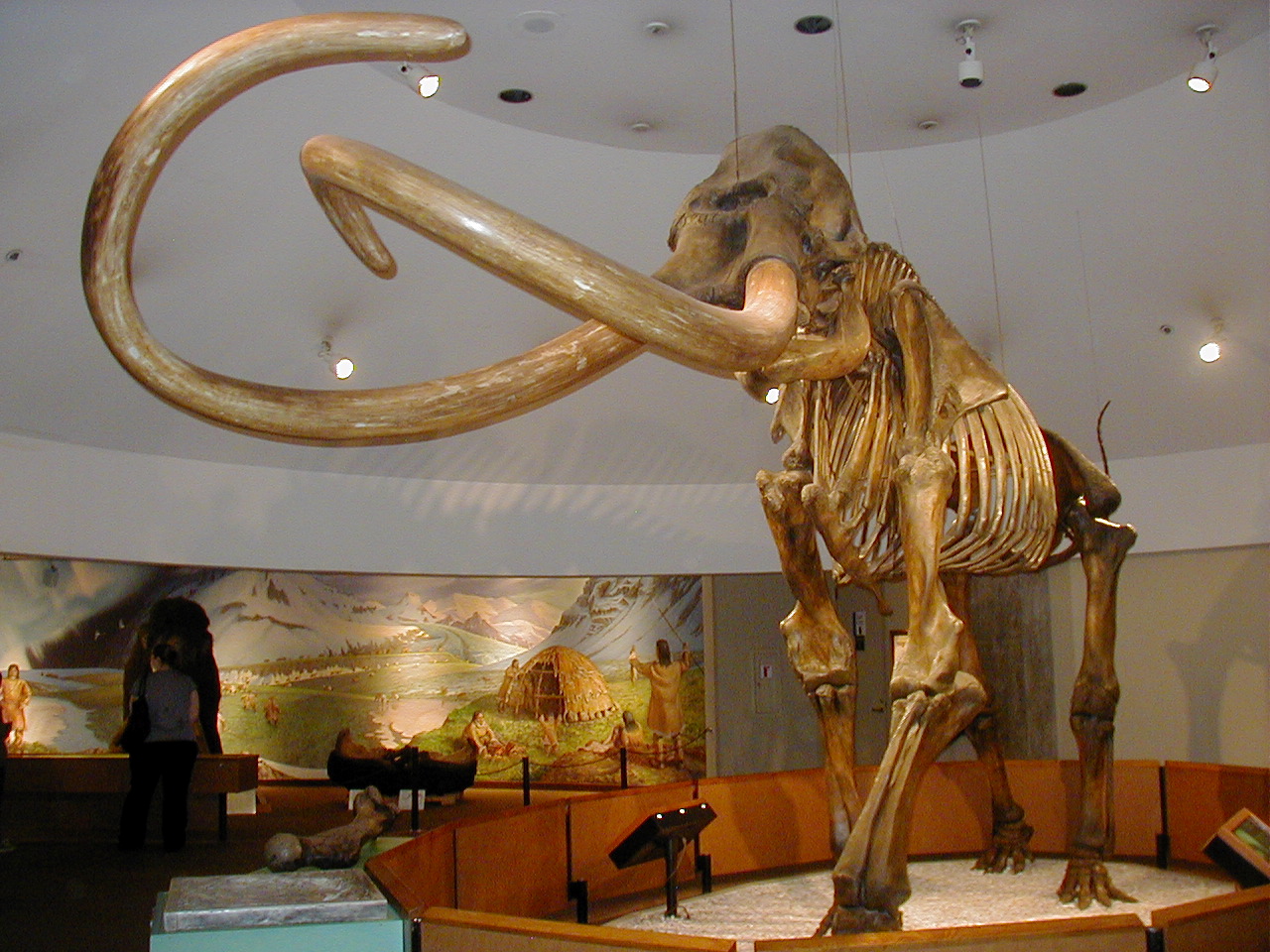The photograph captures the interior of a museum, with the central focus on a massive woolly mammoth skeleton. This impressive display dominates the image, with its long, shiny tusks sweeping to the left. The skeleton, held up by wires connected to the ceiling, features a rusty brown, almost copper color. The ceiling itself is outfitted with numerous lights directed toward the mammoth, illuminating the exhibit despite the overall dim ambiance.

Surrounding the mammoth is a series of wooden barricades designed to keep viewers at a respectful distance. To the lower right of the exhibit, an information display box provides additional context about the mammoth. On the left side of the image, a person can be seen observing another bone display.

In the background, the museum walls are primarily white but adorned with a large mural depicting a scene from an ancient civilization. This artwork features snow-capped mountains, a valley, and people dressed in brown furs, possibly from the Ice Age, gathering around a hut made of sticks. The painting vividly brings history to life, complementing the grandeur of the mammoth skeleton.